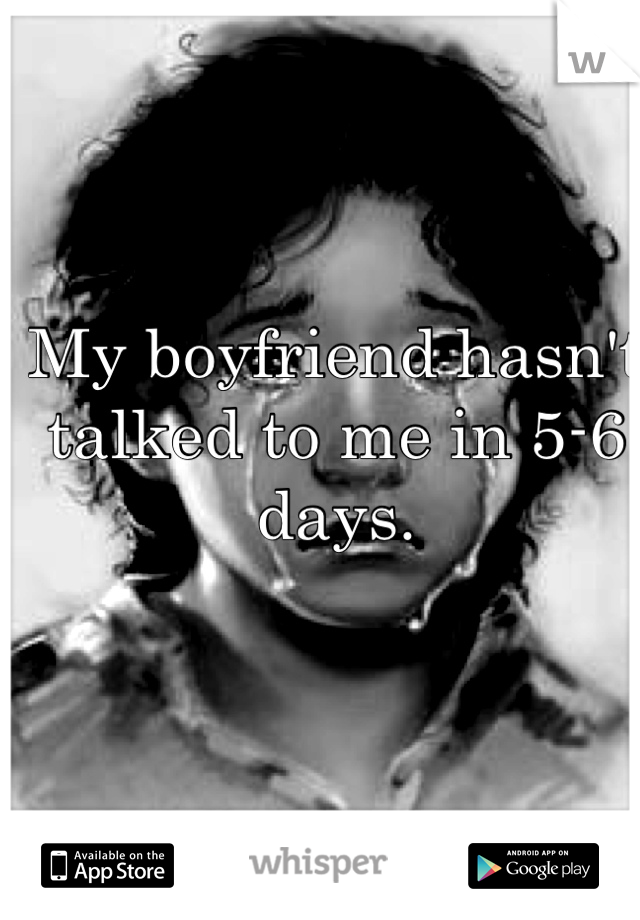This black-and-white image has a digital, meme-like appearance featuring a young woman with medium-length, disheveled black hair and a sad expression. She appears to be crying, with tears streaming down from her eyes to her chin. Her eyebrows are dark, and her collar is slightly askew, revealing her neck. The background is a simple white or gray, intensifying the focus on her emotional state. 

At the center of the image, slightly shifted such that the last letter is off-screen, there's a white text with a black shadow effect that reads, "My boyfriend hasn't talked to me in five to six days." The text is formatted in a basic style. In the upper right corner, there's the letter "W" which stands for Whisper, an app mentioned in the bottom corners of the image. The bottom left features a logo with the tagline "available on the App Store," and on the bottom right, there is a Google Play Store logo with the tagline "Android App on Google Play." Shadow effects around the woman's hair and neck area add depth to the image. Overall, the woman dominates the photo, making her emotional state the focal point.